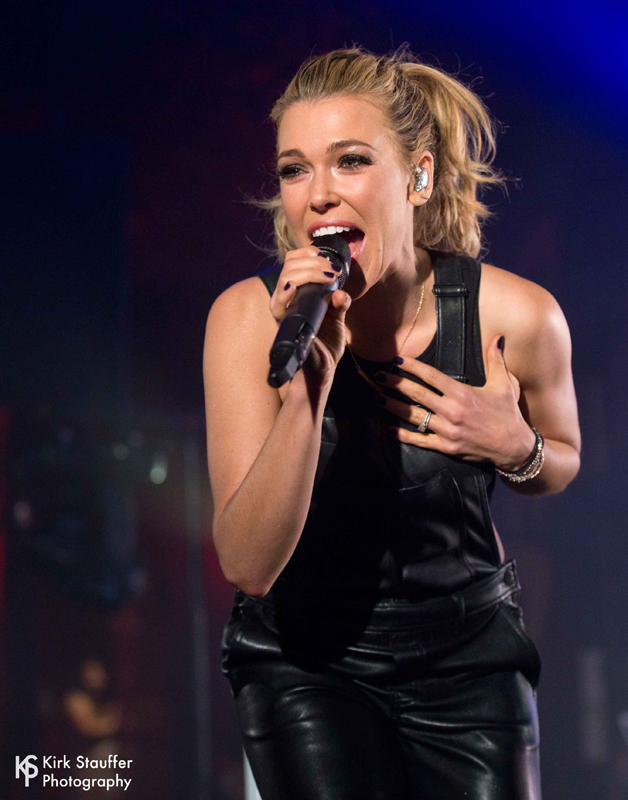The photograph captures a dynamic moment with a Caucasian woman positioned at the center, occupying approximately a third of the frame. She has long, slightly wavy blonde hair styled in a high ponytail, revealing a white earbud in her right ear. Her attire consists of a black, sleeveless, spandex bodysuit, paired with leather overalls. In her left hand, adorned with bracelets and possibly dark red nail polish, she presses her upper chest while her right hand holds a cordless microphone near her mouth. She appears to be singing, her expression a mix of a smile and concentration, with only her top teeth visible. Her body is facing forward, but her head tilts slightly to the left, possibly squinting with minimal makeup.

In the top left corner, the background features a blend of blue and pink tones, transitioning smoothly into one another. Dark blue shapes and clusters of blue and purple lights are discernible along with some peach tones forming a loose triangular shape. The bottom left corner of the photo is marked by a white logo, consisting of a 'K' and an 'S' connected by a vertical line. To the right of the logo, in smaller text, are the words "Kirk Stauffer Photography," with the first letter of each word capitalized. The background in the top right corner fades from a light blue triangular shape into a darker blue. Overall, the image conveys a sense of vibrant energy and artistic expression, enhanced by the branding of Kirk Stauffer Photography.